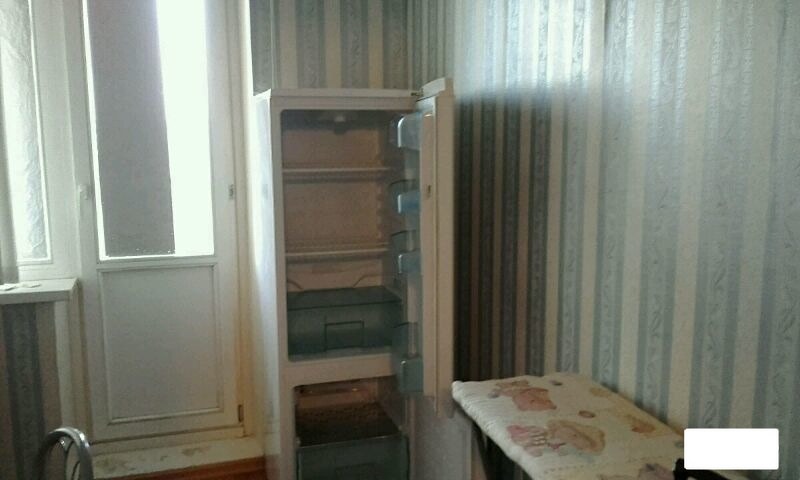The image depicts an indoor kitchen scene characterized by a distinctive blue and white striped wallpaper with intricate swirls and floral patterns adorning the blue stripes. Centered against the back wall is an older style, white refrigerator, its top and bottom doors both open to reveal empty shelves and tinted plastic drawers inside, with no interior light illuminating it. Adjacent to the refrigerator is a door with a window pane leading outside, suggesting daylight. To the left of the refrigerator stands a small, protruding white shelf, and a glimpse of a dark wooden chair with a curved top is visible. The room appears largely empty, with a noticeable lack of furnishings or items on the countertops, and a curiously placed cushioned stool with children and bear patterns adds a touch of whimsy to the stark, utilitarian space.